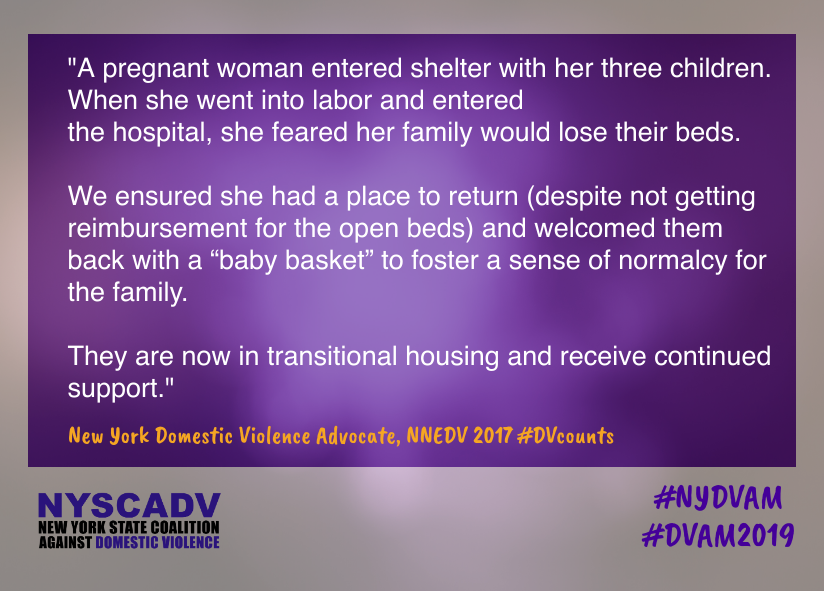A screenshot with a dark purple background displays a heartfelt narrative in white text. It reads, "A pregnant woman entered the shelter with her three children. When she went into labor and entered the hospital, she feared her family would lose their beds. We ensured she had a place to return despite not getting reimbursement for the open beds and welcomed them back with a baby basket to foster a sense of normalcy for the family. They are now in transitional housing and receive continued support." 

Overlaying this narrative, orange letters announce, "New York Domestic Violence Advocate, NNEDB, 2017, #DBCounts." The purple background is framed against a gray backdrop. In the bottom left corner, it is stamped with, "NYSCADV, New York State Coalition Against Domestic Violence," and in the bottom right, "#NYDVAM, #DVAM2019."

The image lacks photographic elements and contains no people, animals, plants, buildings, vehicles, or other common visual subjects. Its focus remains purely on the written text and its impactful message.